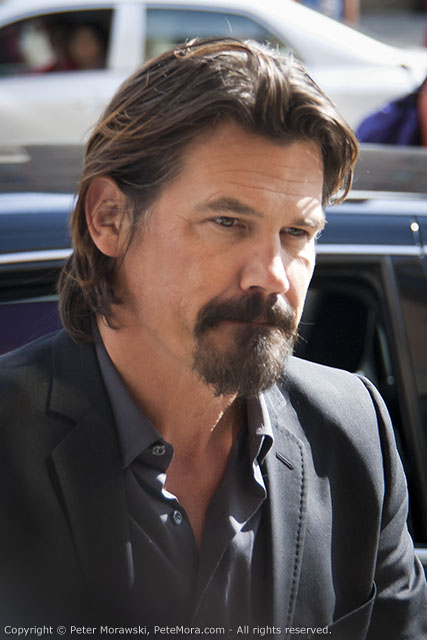This detailed photograph features the renowned actor Josh Brolin. He is dressed in a casual, yet elegant, dark suit paired with a dark shirt that is open at the collar, giving a sophisticated yet relaxed vibe. His brown hair, slicked back and falling to his shoulders, complements his neatly trimmed mustache and goatee. Josh stands centrally in the image, with a neutral yet conscious expression on his face, possibly indicating he is aware of the camera or deep in thought.

In the background, an SUV or limo with a distinctly visible blue roof is parked behind him, while another white car is also noticeable further back. There's a hint of another person in the upper right corner of the photograph, but only their shoulder is visible, adding a subtle layer of complexity to the scene. The bottom of the photo reads "copyright Peter Murawski, Petemor.com, all rights reserved," confirming that Peter Murawski is the photographer. This well-composed photograph captures both the essence of Josh Brolin's casual style and the bustling environment around him.